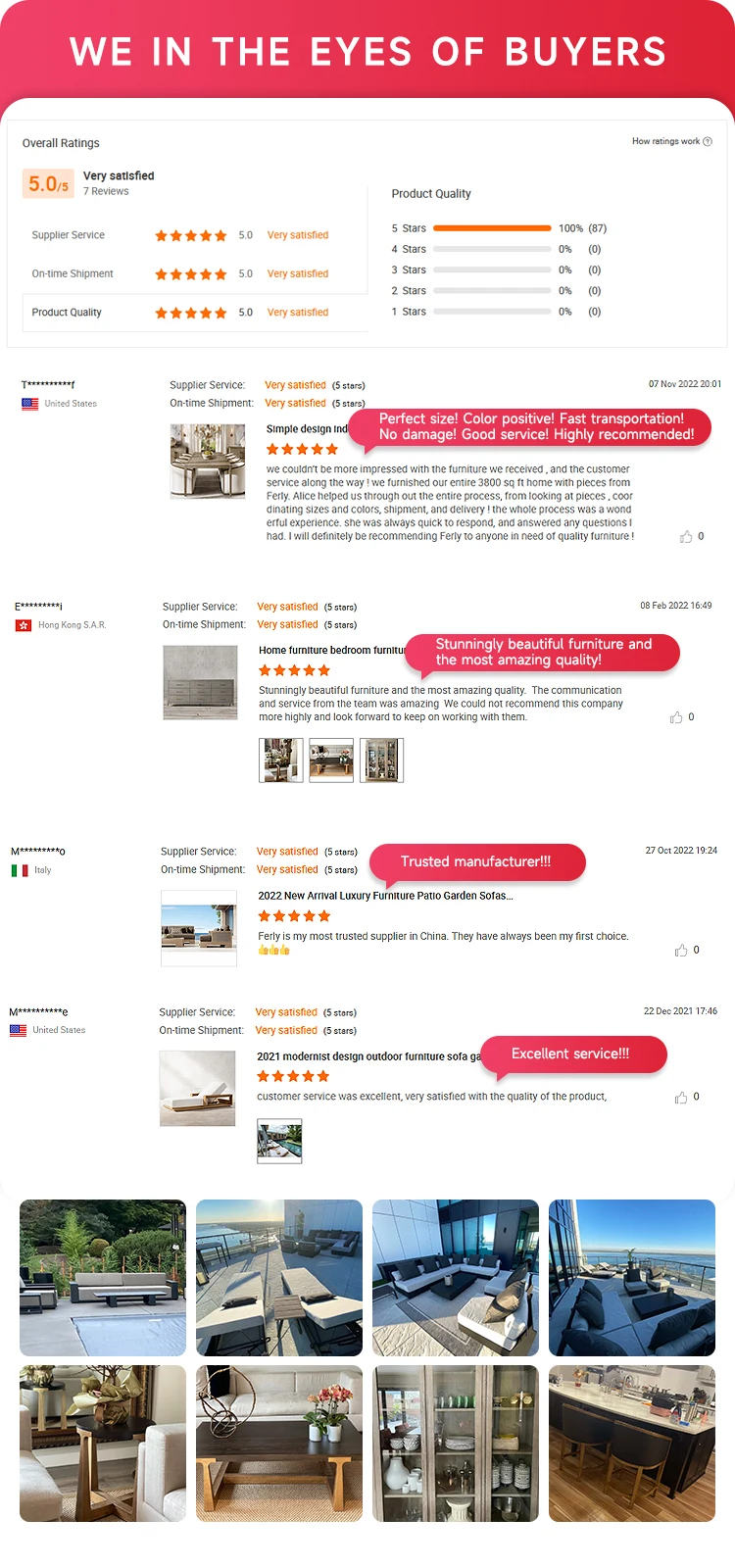A screenshot of a review section on a hotel property review site, displayed in the format of a cell phone screen. At the top of the image is a striking red rectangle spanning the entire width of the screen, with the phrase "We, in the eyes of buyers" written in white letters. While the English here is slightly awkward, it implies feedback from customers. Beneath this heading are four detailed reviews, each paired with small author photos and showcasing consistent 5-star ratings. The reviews vary in length but are uniformly positive. Finally, the bottom portion of the screen is divided into eight photographs. The top row features four images of outdoor furniture arranged on high-rise building decks, offering a glimpse of urban landscapes. The bottom row showcases four different pieces of hotel room furniture, hinting at the property's interior decor.